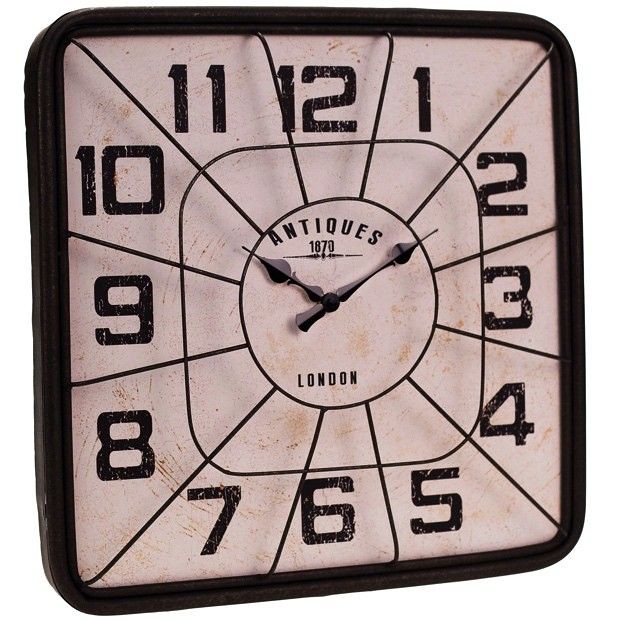The image features a unique, square-shaped antique clock with rounded corners and a black border. A notable focal point is a raised black wire cage over the clock's face, consisting of a central ring with approximately 10 to 11 radiating lines extending to the edges, and visible due to the shadows cast by directed light. The clock's face is a light off-white color, streaked with small, irregular brown and light-colored marks, giving it a worn, aged appearance. Its Arabic numerals, displaying 1 through 12, are in a dark font and also exhibit similar light-colored streaks. The hour and minute hands are black and feature pointed arrows at their ends, currently positioned at 10 and 2, respectively. At the center of the clock, the text reads "Antiques, 1870" with a decorative line below, and "London" beneath the hands. The design and condition of the clock indicate its vintage aesthetic and age.